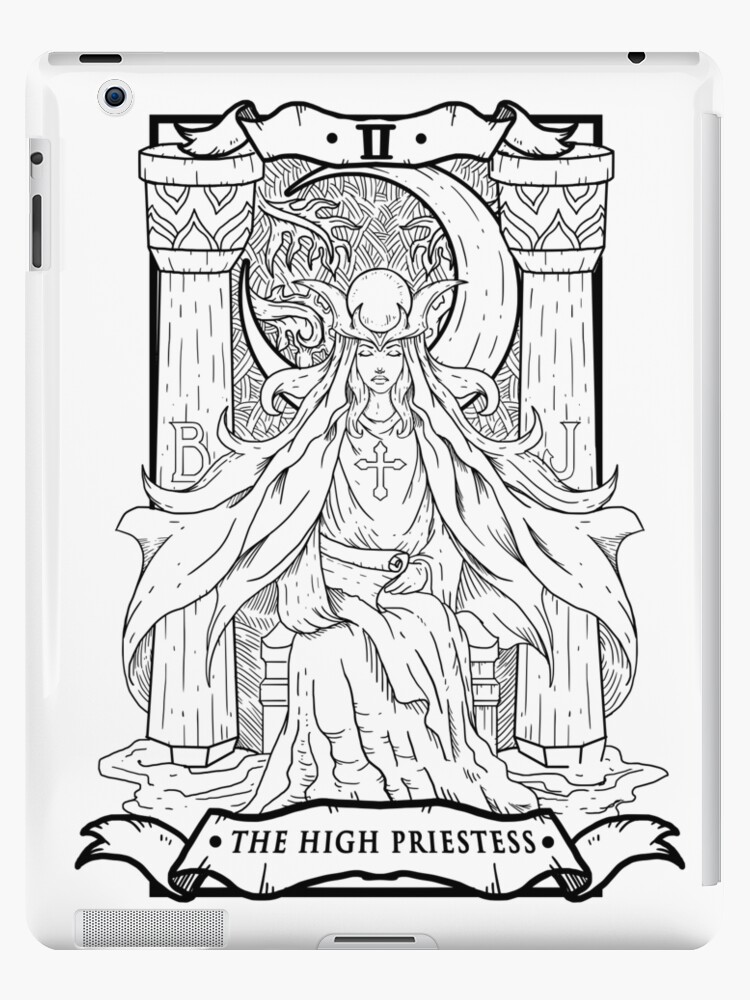This detailed black-and-white drawing, set within a black banner, depicts a woman identified as 'The High Priestess.' She sits regally on a throne, adorned in an elegant gown and wearing a cross necklace prominently displayed at the center of her chest. Her hair is long, and her eyes are gently closed, exuding an aura of serenity and wisdom. Above her, a banner draped across the back of the throne bears the Roman numeral II. The backdrop includes two imposing pillars, each inscribed with the letters 'B' and 'J.' In one hand, she holds a scroll, suggesting her role as a keeper of knowledge. Atop her head, a distinctive white circle crowns her with a traditional regal headpiece, completing her authoritative and mystical appearance. This artwork’s intricate details and symbolic elements suggest it could be part of a game or themed series.